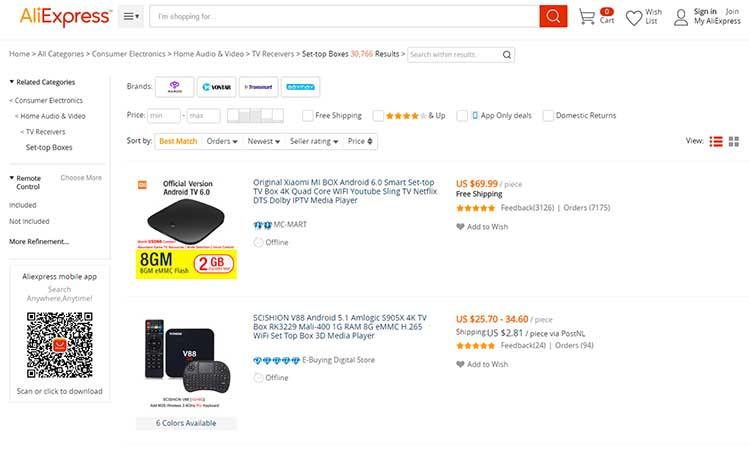The image is a screenshot from the online merchant AliExpress. Across the top, the AliExpress logo is prominently displayed, followed by a search bar, a magnifying glass icon, a shopping cart icon, a like button, and a sign-in button. Just below this, various credit card logos are shown, indicating accepted payment methods.

In the far left-hand corner, there is a navigation menu with related categories such as Consumer Electronics, Home Audio & Video, TV Receivers, and Set Top Boxes. Under these categories, there are further refinements, specifying options like "Remote Control Included" and "Not Included." Additionally, a QR code is positioned below the category list.

To the right, several search filters are available, including options for price, free shipping, ratings of four stars and above, app-only deals, and domestic returns. Sorting options are also provided, allowing users to sort by orders, newest arrivals, seller ratings, and price.

The first product displayed is the "Original XEOMI MI Box Android 6.0 Smart Set Top TV Box." This 4K quad-core device supports Wi-Fi, YouTube, Sling TV, Netflix, DTS, Dolby, and IPTV. The product image shows a sleek black box labeled "Official Version Android TV 6.0," with specifications listing 8GB internal storage and 2GB RAM. The price for this item is $69.99 with free shipping, and it has received a 5-star rating.

The second product featured is the "Scyssian V88 Android 5.1 Amlogic S905X 4K TV Box." This set-top box boasts an RX3229 Mali-400 GPU, 1GB RAM, 8GB eMMC storage, and supports H.265, Wi-Fi, and 3D media playback. The image shows a black box, a remote control, and what appears to be either a keyboard or a game controller. The price ranges between $25.70 and $34.60, with shipping costing $2.81. It also has a 5-star rating, with 94 orders placed, and an option to add the item to a wish list.